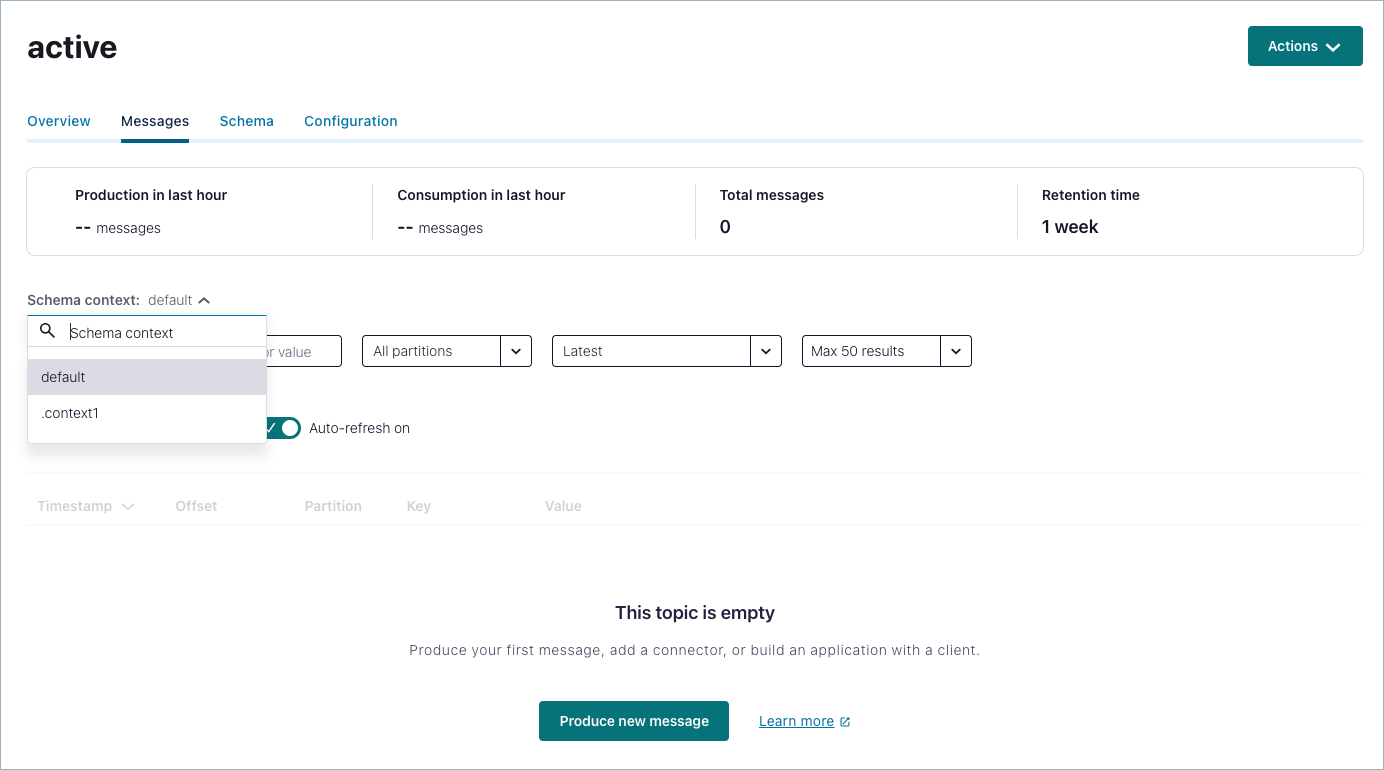The screenshot depicts a web page interface predominantly featuring a white background. 

In the top left corner, the word "active" is displayed in lowercase black letters: "a-c-t-i-v-e". On the far right-hand side, there's a green button with white text that says "ACTIONS" alongside a down arrow, indicating a dropdown menu.

Beneath "active", a blue line spans the width of the page. Directly above this line, in small print, are the labels "OVERVIEW", "MESSAGES", "SCHEMA", and "CONFIGURATION". "OVERVIEW", "SCHEMA", and "CONFIGURATION" are presented in blue, while "MESSAGES" is in dark text with an underline, signifying that the "MESSAGES" section is currently selected.

Below this navigation bar, a box contains several pieces of information organized in rows. The top left corner of the box includes the text "PRODUCTION" and "LAST HOUR". Adjacent to "MESSAGES", it displays: 
- "CONSUMPTIONS" with "LAST HOUR" 
- "TOTAL MESSAGES" with the number "0"
- "RETENTION TIME" of "one week"

Further down, there is a dropdown search labeled "SCHEMA CONTEXT" with options "DEFAULT" and "CONTEXT 1" available for selection. Several subsequent boxes feature dropdown menus labeled "VALUE", "ALL PARTITIONS", "LATEST", and "MAX 50 RESULTS".

At the bottom of the page, a message states, "THIS TOPIC IS EMPTY, PRODUCE YOUR FIRST MESSAGE, ADD A CONNECTOR, or BUILD AN APPLICATION WITH A CLIENT." Below this, two buttons are positioned; a green one that says "PRODUCE A NEW MESSAGE" and another labeled "LEARN MORE".